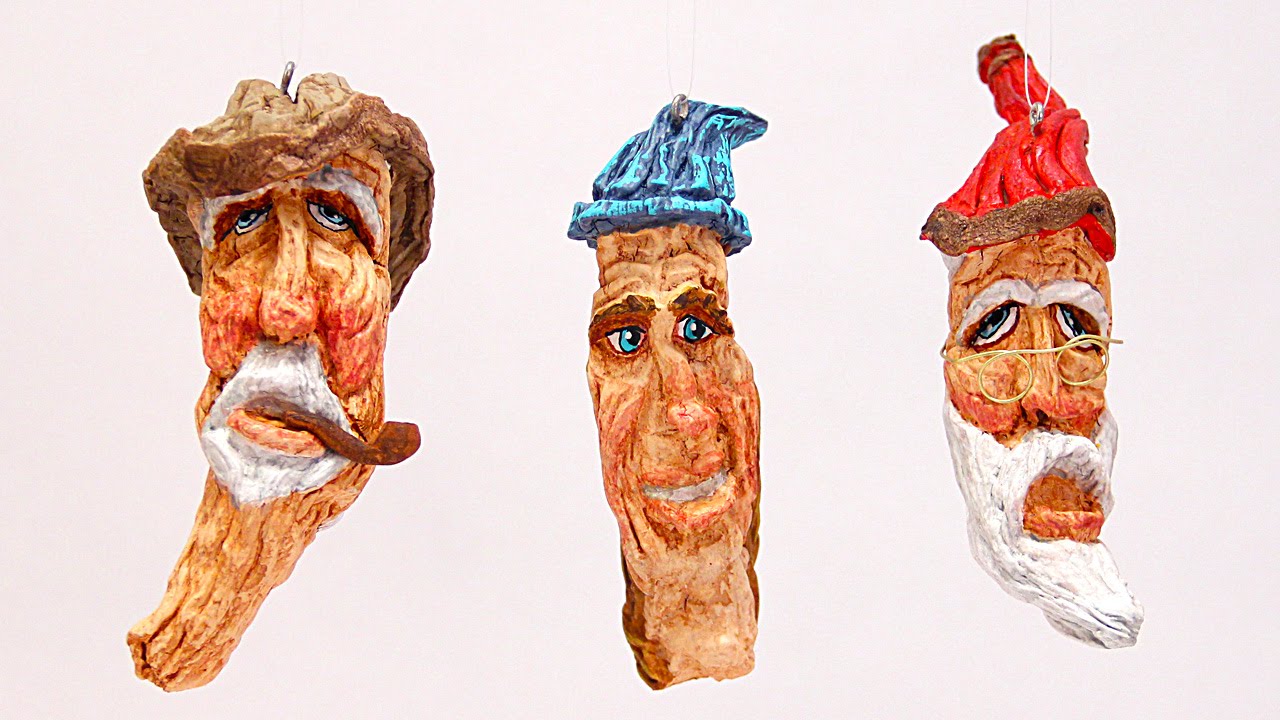This photo showcases three intricately carved wooden ornaments, each presenting the elongated faces of old men, with diverse expressions and distinct details. They hang suspended against a blank background, giving emphasis to their finely crafted features. 

The first figure, on the left, depicts an old man with a white beard and white eyebrows, wearing a brown brimmed hat and rosy red cheeks. His light blue eyes gaze out solemnly, and a pipe extends from his mouth, adding to his wise, contemplative demeanor. The middle figure features a younger man with a cheerful expression. He sports brown eyebrows, medium blue eyes, and no beard. His head is adorned with a blue snowcap that matches his eye color, suggesting a more carefree spirit compared to his counterparts. Finally, the figure on the right represents another elderly man, distinguished by his long white beard, white eyebrows, and numerous wrinkles. He wears gold glasses and a red hat with brown accents. All three figures have small metal hooks fixed to their heads, threaded with white string, emphasizing their status as hanging ornaments and showcasing a blend of artistry and whimsy in their presentation.